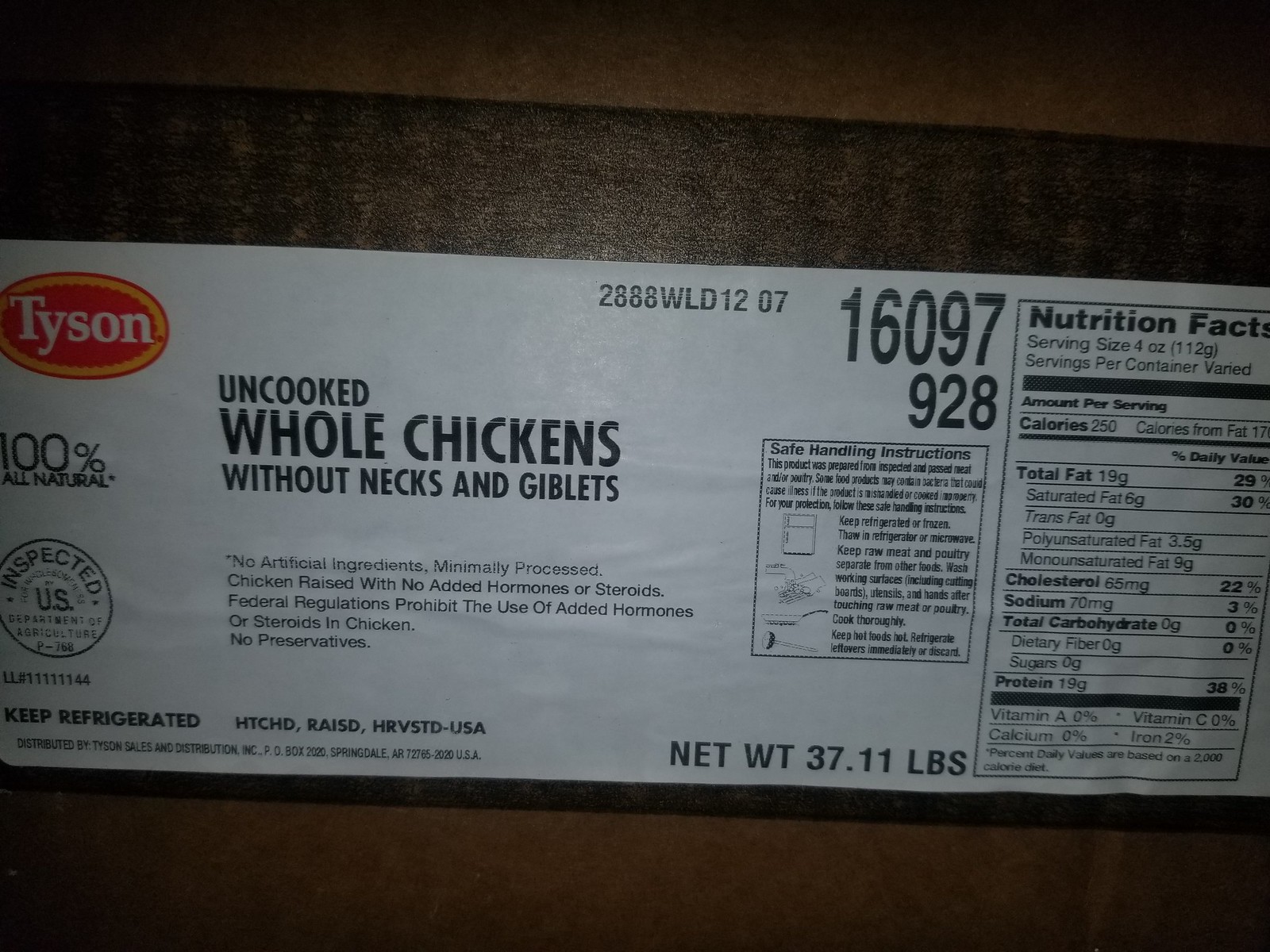This is a detailed photograph of a package of uncooked whole chickens from Tyson, specifically without necks or giblets. The image is in color and landscape orientation, featuring a dark wooden table in the background. The prominent Tyson label is visible, displaying the logo in orange and yellow on the top left corner, with a stamp indicating that the chickens were USA inspected and harvested in America. The label also clearly states "100% natural" and emphasizes keeping the product refrigerated. The total net weight of the package is 37.11 pounds. Nutritional information is detailed on the label, including a serving size of 4 ounces, with varying servings per container. Each serving contains 250 calories, 19 grams of total fat, 6 grams of saturated fat, and zero trans fat. The packaging material appears as a long, narrow strip laid out on the table, encompassing all these details.